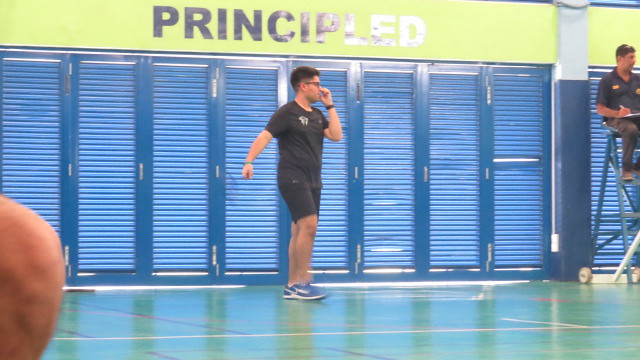The photograph, taken indoors in an arena or sports hall, captures a detailed scene within a rectangular frame that is wider than it is tall. At the top of the image is a yellow or green banner featuring the word "Principled" in bold, dark print. Below the banner are floor-length blue lockers or shutters with horizontal slats, suggesting a wall of shuttered blinds.

In the center stands a man with light skin, short black hair, and glasses. He is dressed in a short-sleeved black shirt, black shorts, and blue and white tennis shoes. His left arm is bent at the elbow, reaching up toward his face, while his right arm extends outward to the side. The area around him features a green floor marked with various colored lines, indicative of a sports court.

On the lower left-hand side, either a thumb or the back of a bald head is partially visible in the foreground. To the right, a man with short brown hair is seated on an elevated overview seat, commonly used for officiating sports like volleyball. He sports sunglasses on his head, a blue polo shirt, black trousers, and holds a clipboard and pen, looking off towards the right side of the image, presumably watching the ongoing activity.